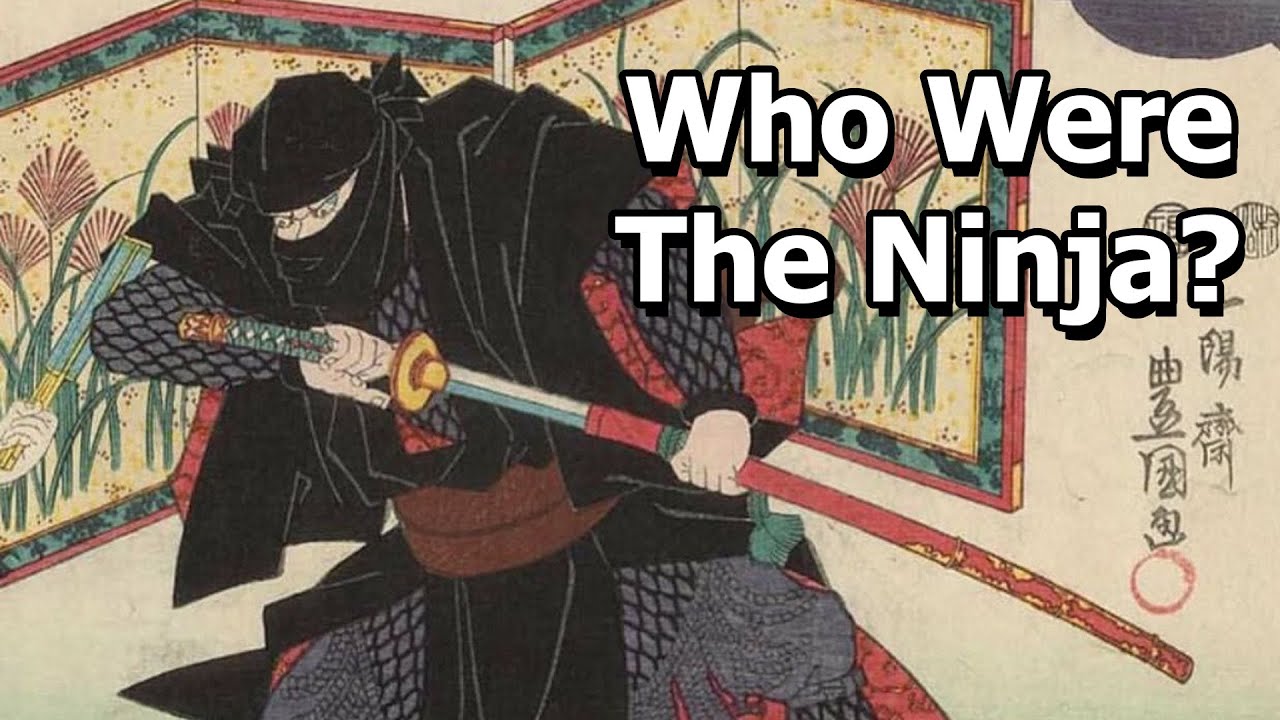This poster features a striking image of a Japanese ninja, dominating the frame, with an imposing text in capital letters on the upper right that reads, "WHO WERE THE NINJA?" accompanied by a question mark. The majority of the background is white, with intricate black Asian lettering adorning a beige wall. The ninja is depicted in traditional attire, wearing a black hood that only reveals his eyes through a crescent-shaped slit, and a black robe tied with a belted tie. His attire also includes chain-link armor in gray, which covers his arms, torso, and legs, as well as black and gray patterned sleeves and pants.

In his left hand, the ninja firmly grips the hilt of an ornate samurai sword. The sword's hilt is detailed with a golden circular piece at the end, leading into a green wrapping near his hand. The blade visible is dark blue and light gray. His right hand holds the sword's sheath, primarily red with gold accents at the bottom and a green section partially hidden by his hand.

The background features a detailed painting with red flowers and green stems, framed by a red leaf embroidery at the top and bottom. This artistic depiction, possibly computer-generated, blends muted colors like salmon, blue-green, and parchment beige, creating a cohesive and historic atmosphere.